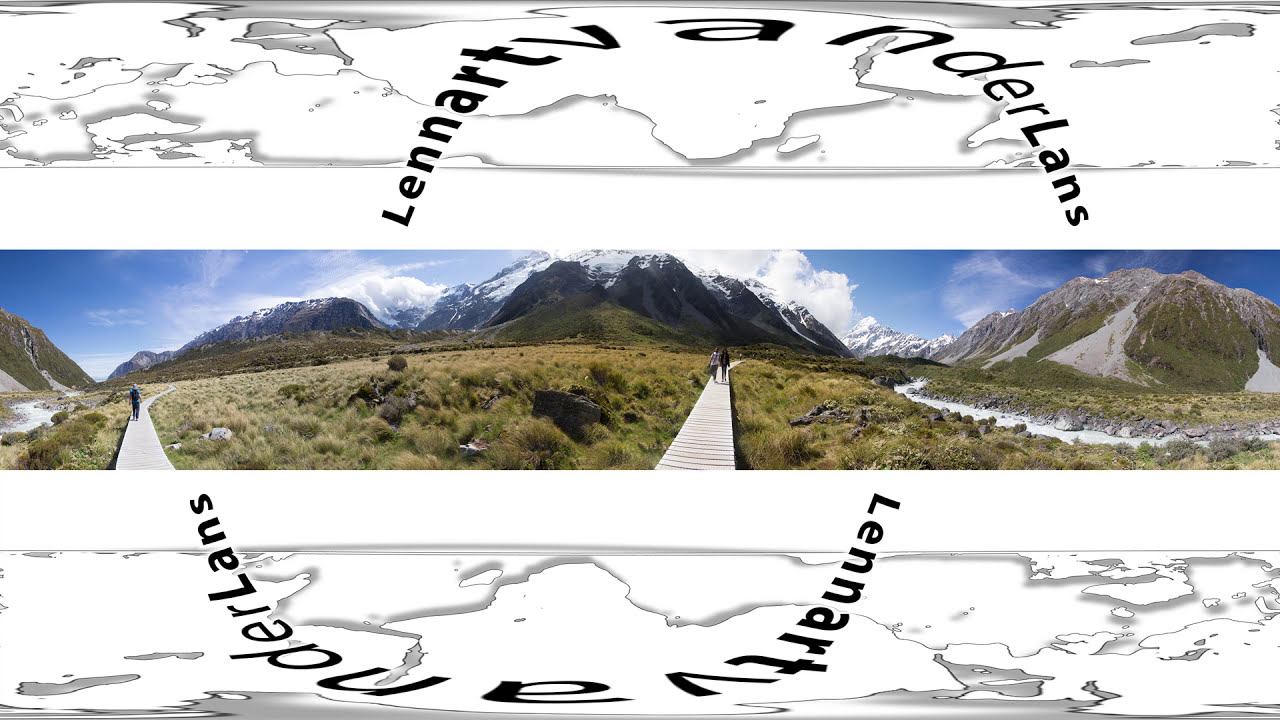The image is a rectangular advertisement featuring a central photograph flanked by computer-generated imagery and text. In the heart of the image, there is a pristine natural scenic view of large snow-capped mountains that span the entire background, with a vivid blue sky dotted by white clouds above them. The foreground of the photograph showcases a lush, rocky landscape with dense greenery, bushes, and grass. Notably, there are two narrow wooden boardwalks or bridges. One bridge runs through the center, leading towards the mountains, inhabited by two people walking in the distance, while the other, to the right, has a single person walking towards the mountains. Flanking these walkways are small, clear streams, enhancing the natural beauty of the scene. Surrounding the photograph, the top and bottom sections feature gray and white, map-like illustrations with the text "Lennart TV Anderlands" in black print. The text on the top is curved upwards, while the bottom text curves downwards, providing a distinct framing for the scenic photograph.